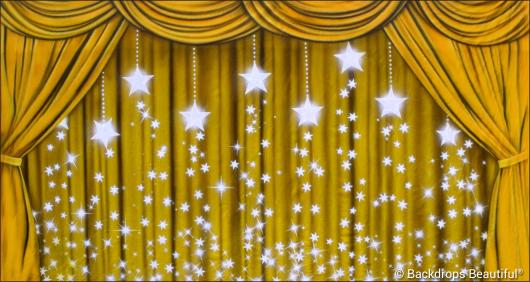This is an image of a stage adorned with light yellow curtains. At the bottom right corner, there is a watermark in small white text that says "Backdrops Beautiful," along with a copyright symbol. The curtains feature four rounded sections at the top, and additional sections are pulled to the sides and held by straps. The foreground is decorated with bright, white shining stars of varying sizes, hanging from small strings attached to the ceiling. The larger stars appear to drop smaller stars like sparkling cascades. Behind the pulled curtains, there is a backdrop of the same yellow color, slightly lighter and wrinkled, running from top to bottom. The arrangement of curtains and the detailed drapery create a brilliant, layered effect that evokes a sense of depth and elegance on the stage.